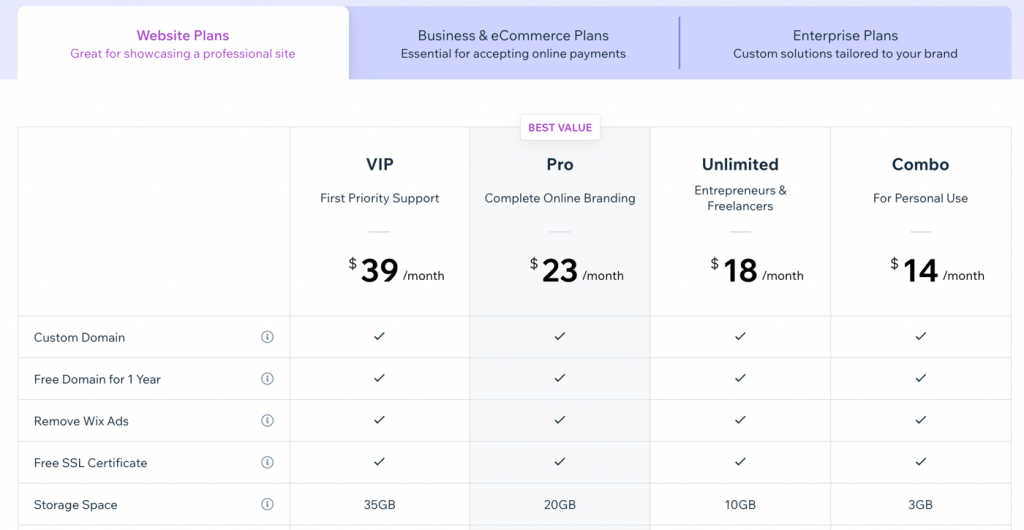This screenshot displays a tabbed interface with a purple navigation bar at the top, showcasing three distinct plans categories: "Website Plans," "Business and eCommerce Plans," and "Enterprise Plans." The "Website Plans" tab is currently selected, indicated by its white background and purple text reading "Great for showcasing a professional site," while the other two tabs are shaded in purple, indicating they are not active.

Below the navigation bar, a comparison graph presents several pricing plans alongside their features. On the left-hand column, the chart lists the features included in each plan: "Custom Domain," "Free Domain for One Year," "Remove Wix Ads," "Free SSL Certificate," and "Storage Space."

The chart details four different plans from left to right: VIP, Pro, Unlimited, and Combo. Each plan is accompanied by a brief description, its respective price, and the included features, represented by checkmarks. Notably, the "Pro Plan" is highlighted with a light gray background and labeled as "Best Value" in purple text. Although all plans include checkmarks for the first four features, the "Storage Space" feature differs, with the VIP plan offering a higher amount of storage.